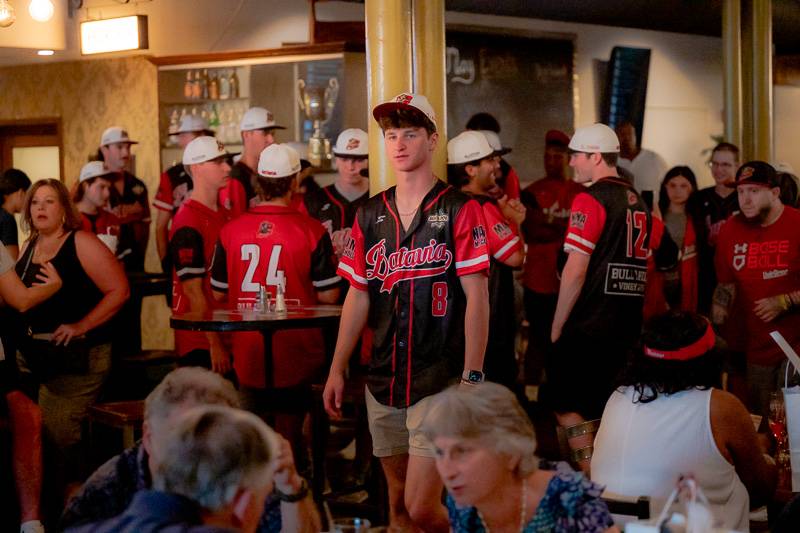In this lively and detailed image, we see the focal point is a central figure in a baseball uniform, wearing a black and red collared jersey that reads "Batavia" with the number 8, paired with khaki shorts. He stands confidently in the middle, looking directly at the camera with a red and white cap on. Surrounding him, several team members can be spotted, all dressed in similar black jerseys with red sleeves and white caps, bearing various numbers like 12 and 24. 

The setting appears to be a bustling restaurant, likely after a sporting event, with multiple conversations happening in the background. To the left and right, groups of people are seated at tables; some have visible salt and pepper shakers on them. Most of the people in the foreground, particularly on the right side, are older with graying hair, engaged in conversations. Among them, different individuals stand out – like an older woman with a black tank top with makeup on the left, and a black woman seen from the back.

The interior décor of the restaurant adds to the vivid scene – there are yellow columns, one prominently in the middle and another on the right. The back wall features an old-style wallpaper, a trophy, and shelves with bottles. On the right, a large blackboard with white writing is visible, adding a nostalgic touch to the atmosphere. The lighting in the space includes a square light in the upper left corner and two round lights, along with an oval light, illuminating the animated gathering.